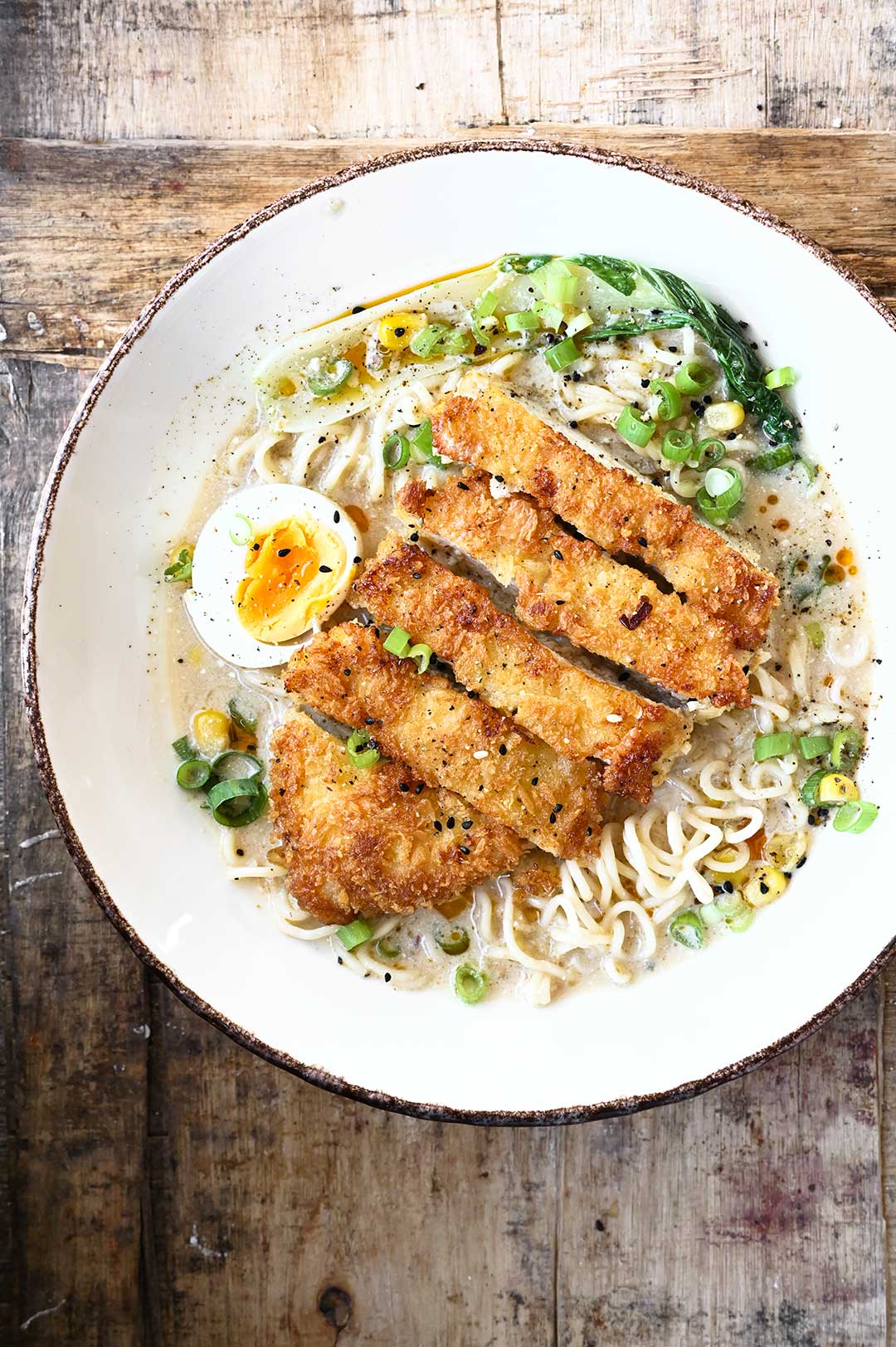The image shows a beautifully presented noodle dish, served on a plate that is round and ivory white with a sponged brown rim. The plate is positioned on an old, worn, light-colored wooden table, giving it a rustic charm. The dish features ramen noodles submerged in a rich broth, topped with a variety of ingredients. At the center of the plate lies a breaded and fried cutlet, sliced into five crispy golden-brown pieces, likely chicken or pork. Surrounding the cutlet are finely chopped green onions, black sesame seeds, kernels of corn, and what appears to be a mix of green vegetables such as spinach. To the left side of the cutlet, there is half of a soft-boiled egg. The visually striking combination of colors and textures in the dish makes it as appealing to the eyes as it likely is to the palate.